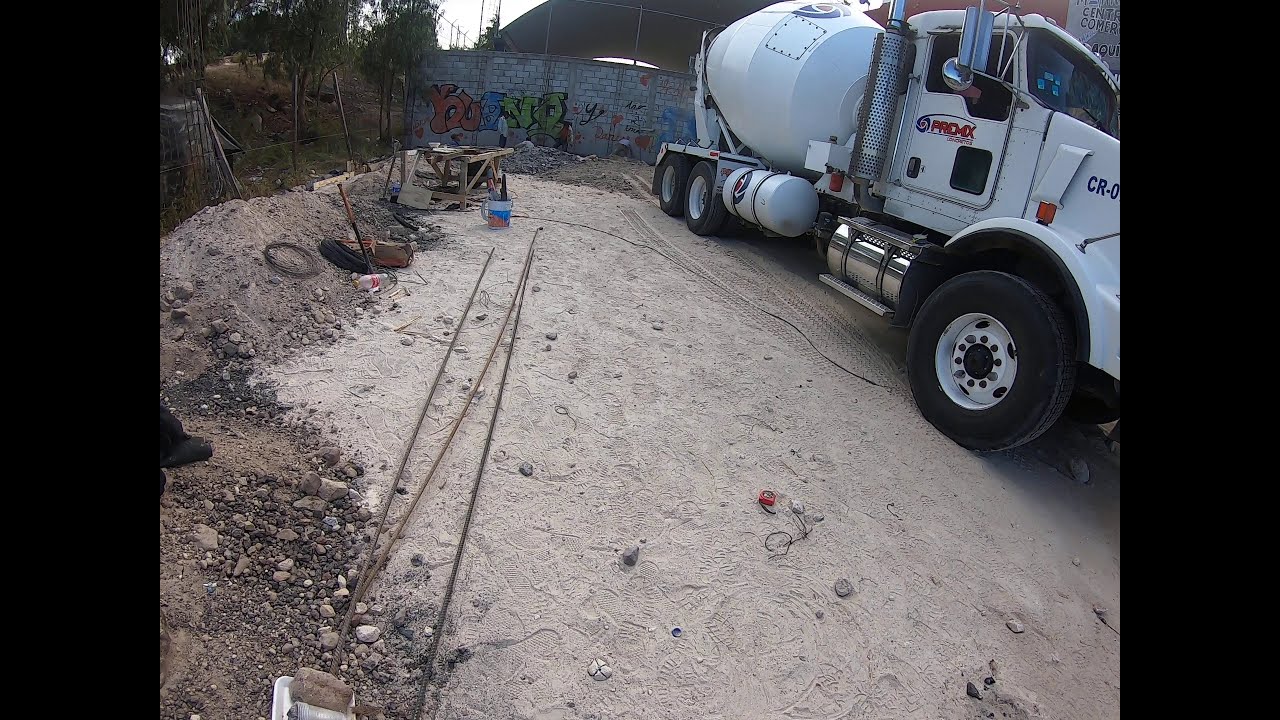The image depicts a white cement truck positioned in the top right corner of a rectangular photograph, framed by tall black rectangles on either side. The truck, bearing the company name "PROMX" in red font on the door and a blue and red logo on its round mixer, is parked in a dirt parking area. It is surrounded by piles of dirt, rocks, and debris such as rebar, suggesting an active construction site or cleared land. The bottom half of the image is dominated by a light sandy patch, while the background features a gray wall adorned with graffiti. Additional structures, possibly a bridge or overpass, and faint figures of workers can be seen in the distance, contributing to the impression of an industrial or construction environment.